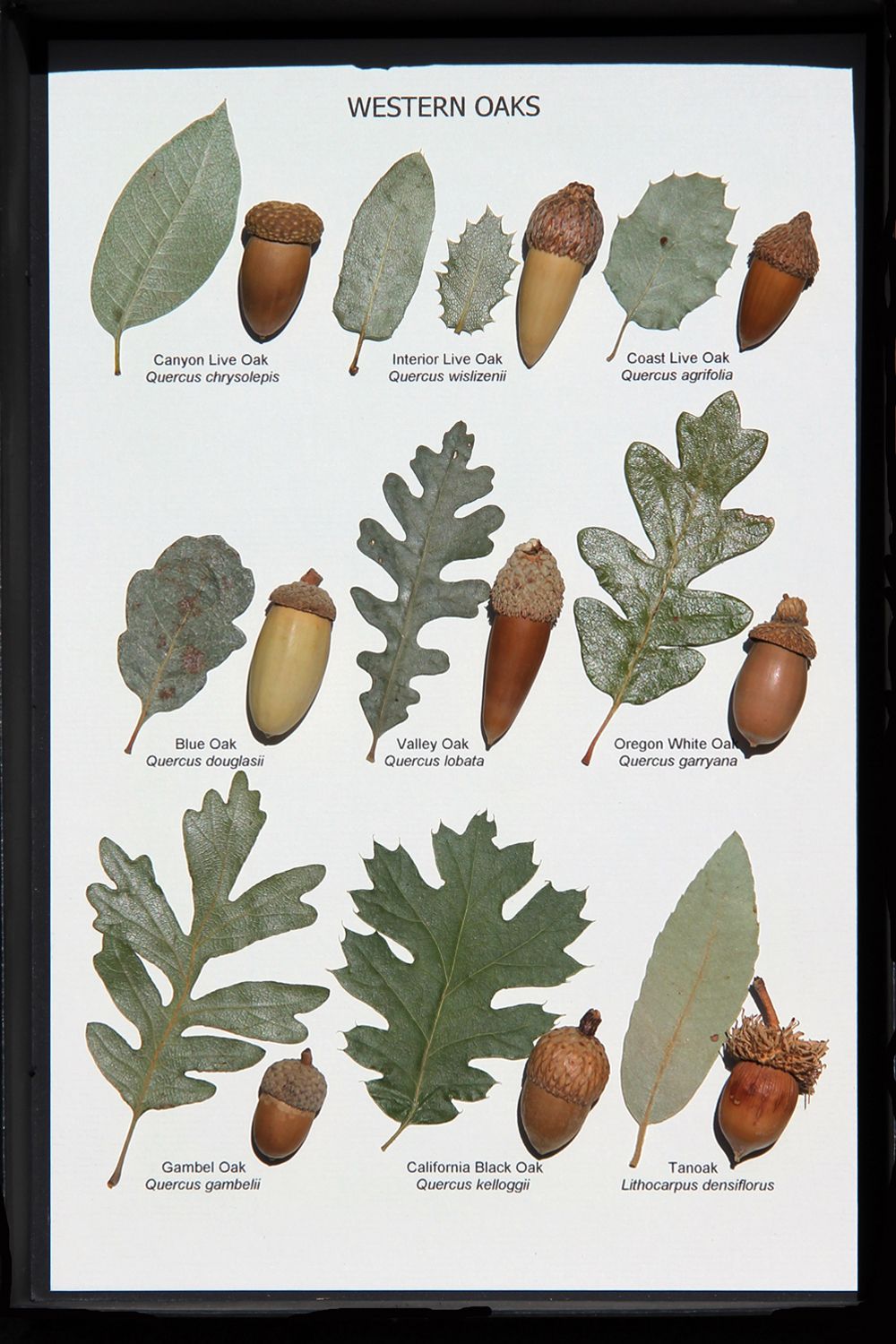The poster, framed in a black rectangular border, showcases a detailed diagram of various leaves and acorns deposited by Western Oak trees, titled "Western Oaks" in small black letters at the top against a white background. The layout includes three columns and three rows, displaying nine different categories of oak leaves and their corresponding acorns. Each category identifies a specific type of oak—such as Canyon Live Oak, Interior Live Oak, Coast Live Oak, Oregon White Oak, Valley Oak, Black Oak, Gamble Oak, California Black Oak, and Ten Terchuk Oak—beneath which the respective leaf and acorn are depicted. The leaves vary in shades from light green to grayish, each accompanied by acorns of different shapes and sizes, ranging from tubular to ice cream cone-like forms. In the lower right corner, a notable oak has a light gray leaf paired with a brown acorn featuring a fluffy cap and a protruding stem. The detailed illustrations highlight the variations in leaf shapes—some smooth and some with petal-like structures—showcasing the diversity among Western Oaks.